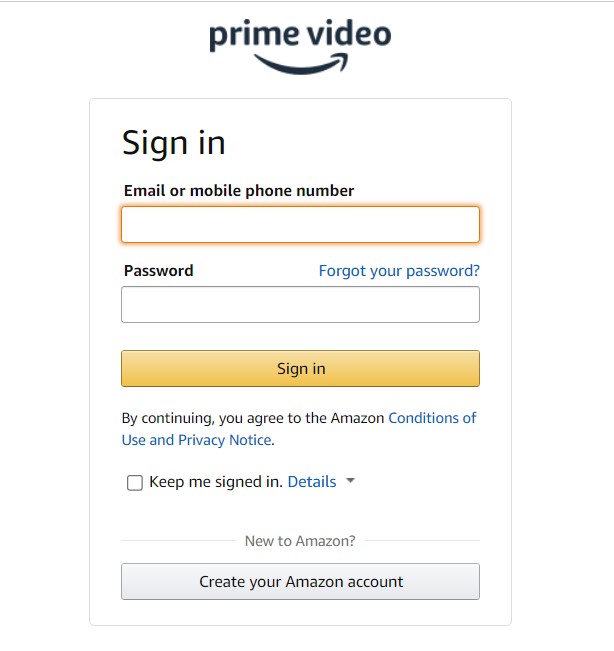This image captures a screenshot from the Prime Video website or app, showcasing the sign-in screen. At the very top, the title "Prime Video" is displayed in black, lowercase print. Beneath this title, a curved arrow arcs from the "I" in "Prime" to the "D" in "Video."

Below the title and arrow, there is a tall, rectangular text box with the heading "Sign in." Directly beneath, it prompts users to enter their "Email or mobile phone number," accompanied by a highlighted entry box with a yellow outline indicating where users should input their details.

Further down, on the left side, there is a label indicating "Password," and on the right side, a blue button labeled "Forgot your password" for those needing assistance with their credentials. Beneath this section, a password entry box allows users to type in their password.

The next section features a rectangular yellow button with black text that reads "Sign in." Below this button, a statement informs users that "By continuing, you agree to the Amazon conditions of use and privacy notice."

Towards the bottom of the screen, there is an option labeled "Keep me signed in" with a small checkbox to its left, allowing users to stay logged in on their device. To the right of this checkbox, the word "Details" appears, accompanied by a dropdown menu for further information.

Finally, the screen addresses new users with the text "New to Amazon?" followed by a gray button labeled "Create your Amazon account," encouraging new users to register for an account.